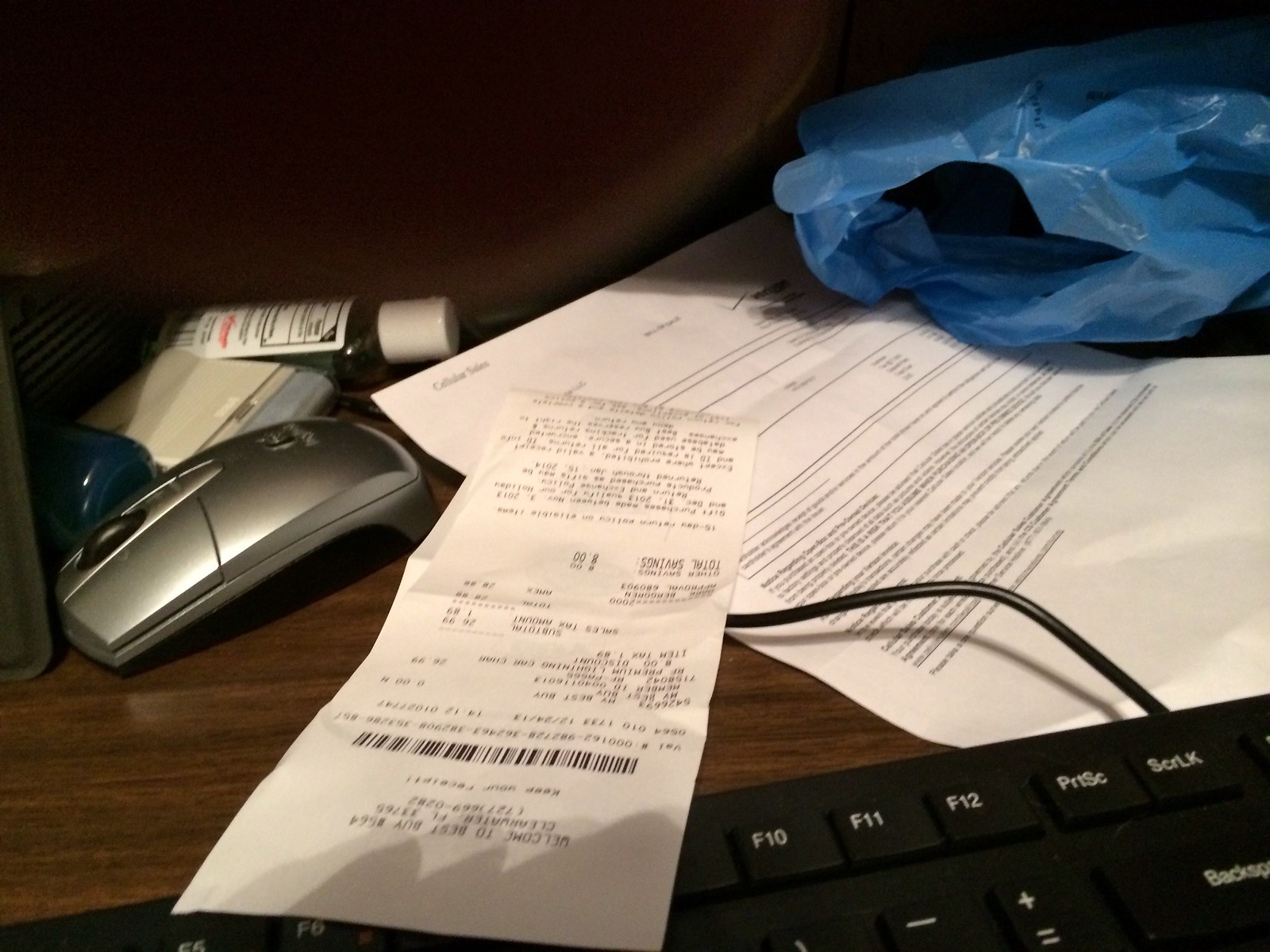This is a photograph of a somewhat cluttered desk featuring a dark to medium brown wooden surface. Dominating the bottom of the image is a black keyboard, partially obscured by a long, shadowed, upside-down white receipt. The keyboard spans from around the F5 key to just past the F12 key, with a visible black wire extending from it, weaving underneath the receipt. Directly to the left of the keyboard lies a silver computer mouse, its top faces the left of the image and it has a black scroll button and black base. Behind the mouse, there's a small bottle, likely containing hand sanitizer, with a white cap and a white label. Adjacent to this bottle is another unidentified dark blue bottle and some sort of gray plastic container. Situational in the upper right-hand corner is a crinkled blue plastic bag, its contents unclear. Sprawled across a significant portion of the desk’s surface, beneath the plastic bag, is a diagonal eight-and-a-half-by-eleven-inch white piece of paper filled with densely packed black text, possibly a statement or document.